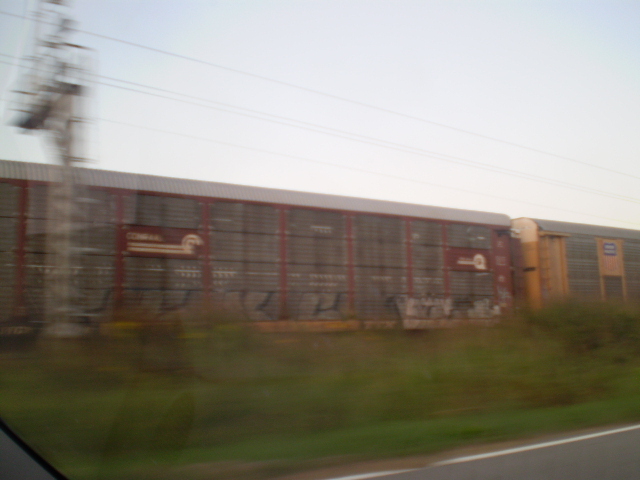This color photograph, taken from a moving vehicle likely through a windshield, captures a blurred scene of a wide, grey building that spans the entire width of the image. The building is prominently featured in the center and has several red columns and two red, horizontally-oriented signs with unreadable white text. Towards the right, there are notable details such as an orange pipe and doors, and a blue sign with white writing at the far right edge of the structure. In front of this building, there is a green, grassy area that is also blurred.

To the left side of the image, there is a thin tower or scaffolding with multiple power lines extending across the sky, which is a gradient of greyish to bluish hues, suggesting it might be either early morning or late evening. Additionally, there is a black asphalt road with a white stripe along the edge at the bottom corners, with hints of a grey and black triangle in the lower left, possibly part of the vehicle's interior. The scene also shows a train track beside the road with visible train cars—one being a dirty brown boxcar with unreadable white text and a logo, and another yellow carrier car ahead of it. Both vehicles and train components contribute to the dynamic and somewhat industrial atmosphere captured in this fleeting moment.